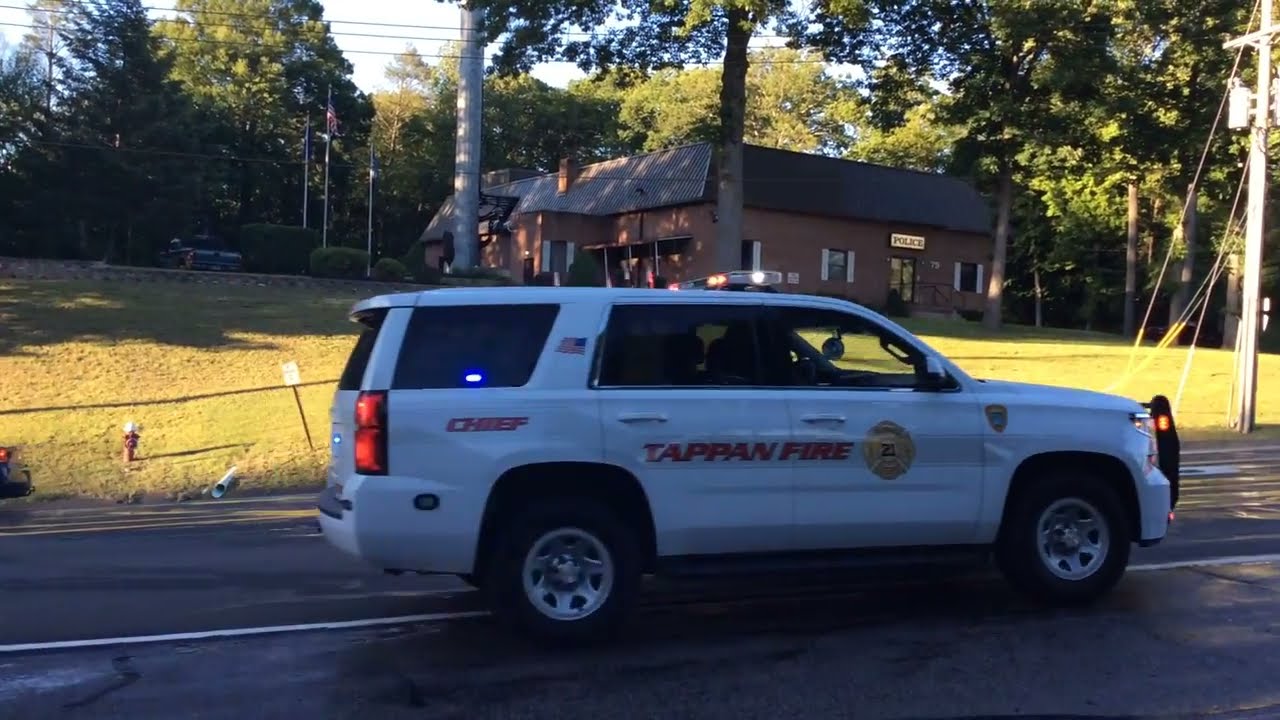The photograph captures a scene on a wet, likely residential, two-lane road. In the center of the image, a white SUV with silver rims and black tires is either moving or stopped, with its brake lights on. The SUV prominently features "Tappan Fire" in red, bold, italicized capital letters on its side, accompanied by a gold firefighter's department emblem. Additionally, "Chief" is written in red letters on the back. There's a USC flag toward the rear of the vehicle.

Behind the SUV, on the side of the road, a large expanse of green grassy field stretches out, bathed in sunlight. Sitting slightly uphill is a brown building with a dark gray or black roof, which appears to be a police station, as indicated by an illuminated sign reading “Police.” Surrounding the building are numerous trees. An American flag is also visible on a pole in this verdant backdrop under a bright, partly white sky.